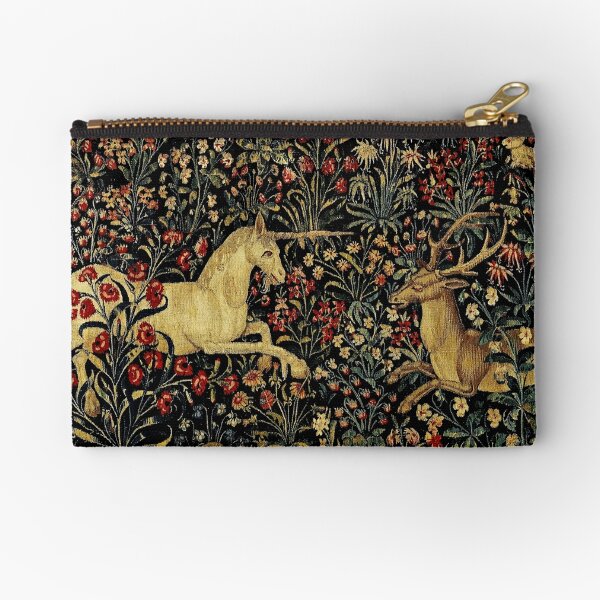This photograph features a highly detailed, small coin purse displayed on a plain white background. The purse, which appears to have been intricately hand-stitched, is adorned with a beautiful tapestry design set against black fabric. Dominating the scene are two fauna figures, a white unicorn on the left, with its horn pointed toward a deer, and the deer on the right, eyes closed and seemingly at peace. The animals, which evoke a vintage, old-timey aesthetic, appear to be lying down in a field brimming with various flowers, including poppies, zinnias, daisies, and other blossoms in reds, whites, pinks, and yellows. Lush green leaves also accentuate the floral landscape, adding to the enchantment of the scene. The purse is functional yet ornate, completed with a gold zipper along the top.